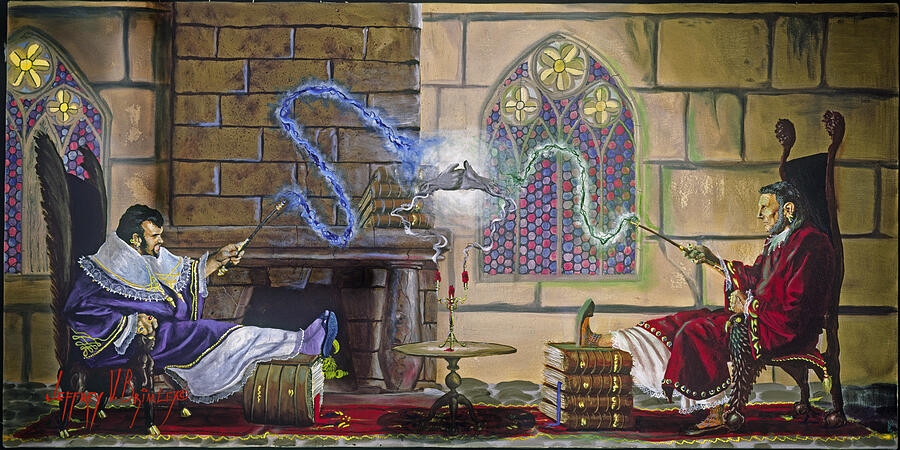The painting, created by Jeffrey V. Brimlexe, depicts a detailed and ornate scene set in what appears to be a castle interior bathed in daylight. The artwork showcases two wizards, seated across from each other in regal chairs, engaged in a magical duel or game. Both men, mirroring each other's posture, have their feet propped up on objects that resemble stacked books or ottomans styled to look like books. 

The wizard on the left sports a black beard and black hair, donning a purple robe embellished with yellow details over a white tunic, and is wearing blue shoes. He is seated in a feathered black chair with a wand emitting a bluish light. The wizard on the right, an older man with a beard reminiscent of Abraham Lincoln, is clad in a red robe over a long white tunic. He reclines in a similarly ornate chair, with his foot resting on an object that looks like a stack of four thick books, and his wand emits a green light. 

Between them, the beams of magic from their wands converge to form two grayish, spectral hands engaged in a thumb war. Below this magical display is a low table adorned with a gold candelabra holding red candles. The background features a brick wall with stained-glass windows in blue, red, green, and yellow floral patterns, adding a colorful and medieval atmosphere to the scene.